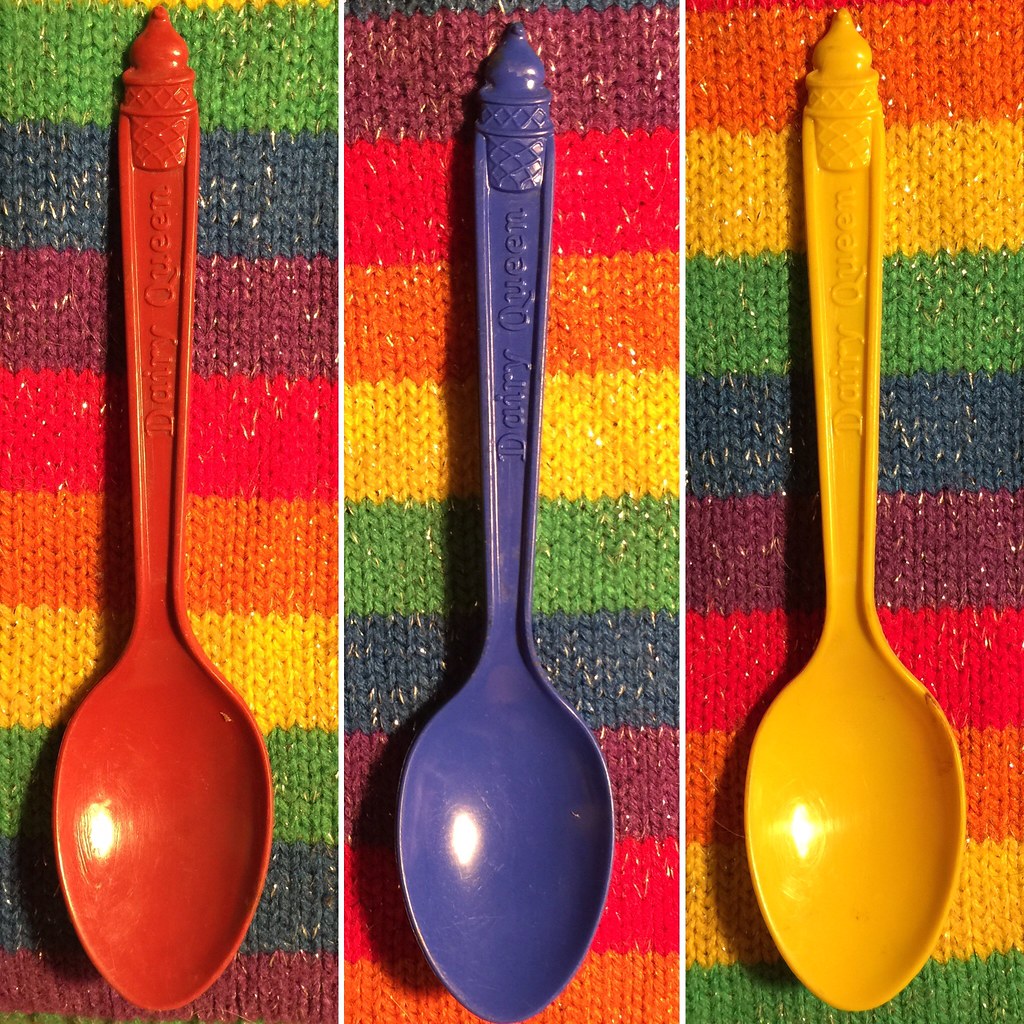This vibrant image showcases three distinct photographs aligned side-by-side, separated by thin white lines, creating a unified, colorful composition. Each photograph prominently features a vertically positioned Dairy Queen plastic spoon set against a rainbow-striped, crocheted fabric background. The spoons, detailed with the Dairy Queen logo and a molded ice cream cone at the handle's tip, vary in color: the leftmost spoon is red, the middle one is blue, and the rightmost is yellow. The crocheted fabric exhibits a repeating pattern of horizontal stripes in green, blue, burgundy, red, orange, and yellow, adding a rich texture to the composition. The spoon tips touch different colored stripes: the left spoon on a purple stripe, the middle on an orange stripe, and the right on a green stripe, collectively enhancing the visual harmony of the image.